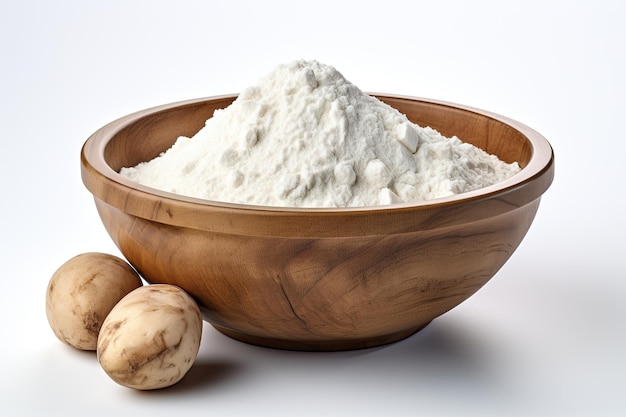In the center of this photograph, a handcrafted wooden bowl with a small lip at the top holds a white, powdery substance that appears to be flour or a similar starch. The flour is mounded into a dome-like shape, peaking in the middle and showcasing some clumps amidst its fine texture. The bowl, made from darker-stained wood, is positioned on a plain white background, accentuated by simple shadows. To the left of the bowl, two medium-sized, slightly immature russet potatoes rest side by side, casting soft shadows. The image has a clean, stock photo feel, meticulously lit from multiple angles, giving it an almost surreal quality.